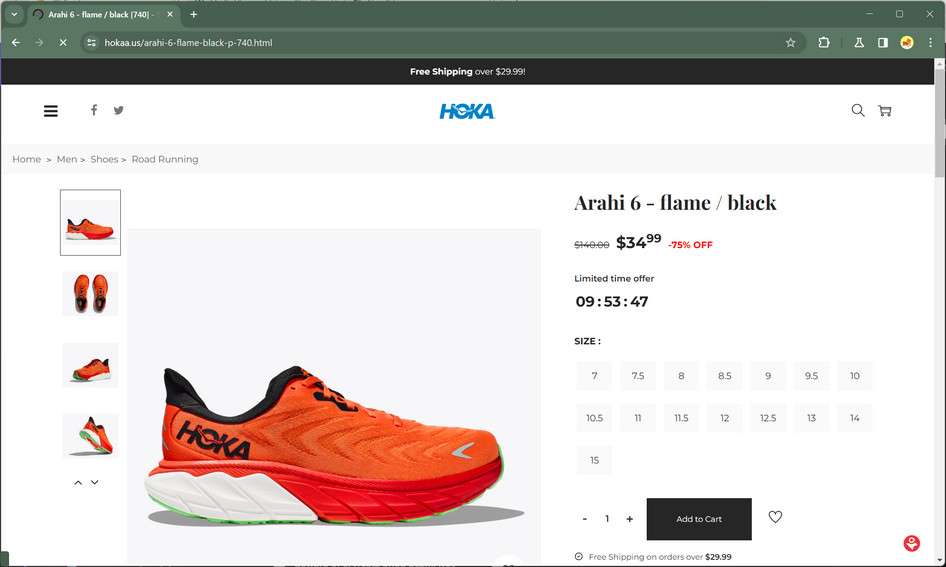This image showcases a website with a layout and design focused on promoting a specific product. At the very top, there's a green grape-colored banner that includes the address bar, which prominently displays the website URL. To the left of the address bar, there are navigation icons: a bright white left arrow key, a faded right arrow key, and an 'X' symbol, also in bright white.

Beneath the address bar, a black banner announces a promotion with the text "FREE SHIPPING OVER $29.99!" in bold, white letters, highlighting the free shipping offer.

The main section of the webpage features a white background with several key elements at the top. On the left, there's a stack of three horizontal lines indicating a menu, followed by icons for Facebook (represented by an 'F') and Twitter (represented by a bird). In the center, the brand name "HOKA" is displayed in capital letters and blue font. To the right of the brand name, there are icons for a magnifying glass (likely indicating a search function) and a shopping cart.

Below this header, the navigation bar includes links such as "Home," "Men," "Shoes," and "Road Running." Along the side, there are four square images stacked vertically, showcasing different angles of the product. The main product display at the center-right side features a shoe with vibrant orange coloring, a white sole, and black trim at the ankle. The text next to the product reads "ARAHI 6 / FLAME / BLACK" with the price listed as "$34.99," showing a significant discount of 75% off.